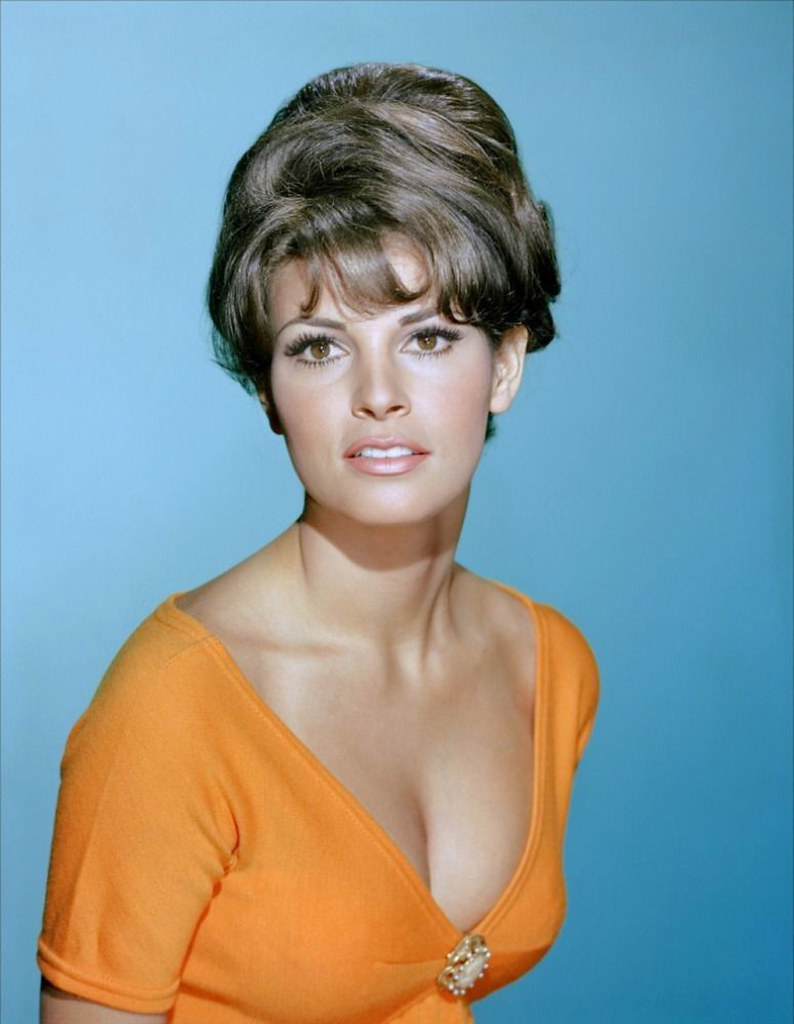The photograph features a woman with brunette hair styled in a vintage, 1950s-inspired updo, including distinct bangs, and her hair is tied up in a bun towards the top of her head. She gazes directly towards the camera, her expression neutral with her head turned slightly to the left. Her brown eyes are accentuated by her slightly parted lips, adorned with light pink lipstick that reveals her upper row of teeth. The woman is wearing a low-cut orange blouse with short sleeves that reach halfway down her biceps. This blouse prominently displays her cleavage and is adorned with a detailed, bejeweled clasp resembling gold and pearls at the center of her chest. The backdrop is a gradient blue, lighter at the top and transitioning to a darker shade at the bottom, creating a subtle, almost shadowy effect.